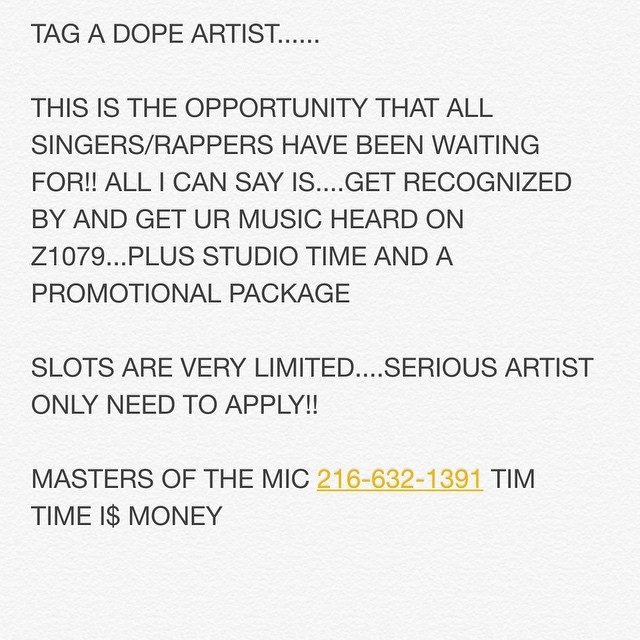This is a photographed image of a typed text message on white paper, presented in capital black letters. The message reads: "TAG A DOPE ARTIST. THIS IS THE OPPORTUNITY THAT ALL SINGERS/RAPPERS HAVE BEEN WAITING FOR. ALL I CAN SAY IS, GET RECOGNIZED BY AND GET YOUR MUSIC HEARD ON Z107.9 PLUS STUDIO TIME AND A PROMOTIONAL PACKAGE. SLOTS ARE VERY LIMITED, SERIOUS ARTISTS ONLY NEED TO APPLY. MASTERS OF THE MIC, PHONE NUMBER 216-632-1391, TEAM. TIME IS MONEY," where the 'S' in "IS" is stylized as a dollar sign. Nothing else is written on the paper.